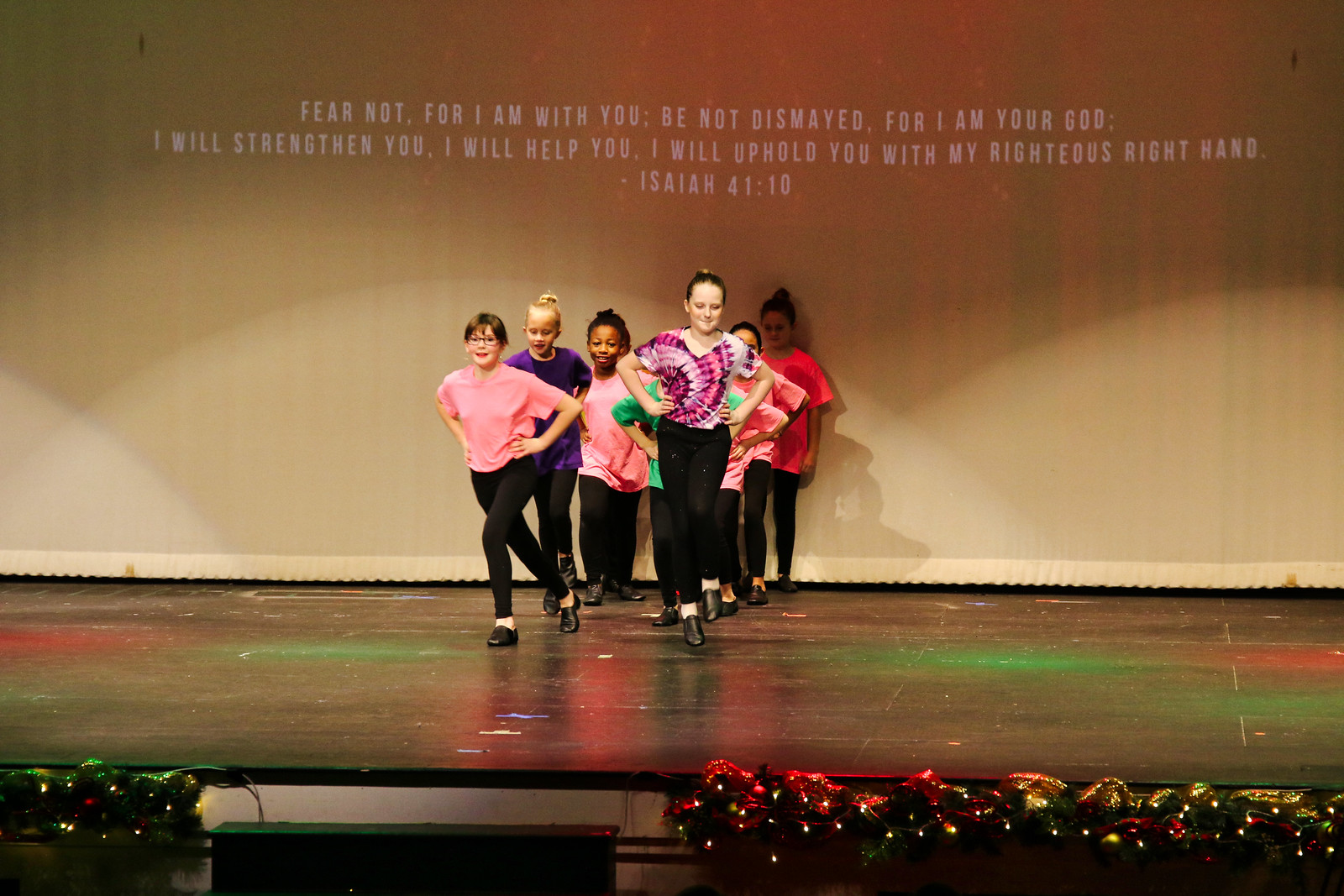In this vibrant image, six children of various ages and races are captured mid-motion during a dance recital, likely held in a church or religious school setting around Christmas time. The group is centered on the black stage, set against a festive backdrop. The stage is adorned with sparkling Christmas decorations, possibly including bows and foliage, illuminated by red and green lights. The children are dressed in a colorful array of purples, pinks, reds, and greens, complemented by black dress pants and stage lights. They wear ballerina-like shoes, enhancing the sense of a spirited performance. Behind them, a back screen wall prominently displays a comforting biblical text in white: "Fear not for I am with you, be not dismayed for I am your God. I will strengthen you, I will help you, I will uphold you with my righteous right hand. Isaiah 41:10." The entirety of the scene echoes the warmth and joy of a holiday-themed talent show, with a beautifully decorated stage juxtaposed against a tan back wall.